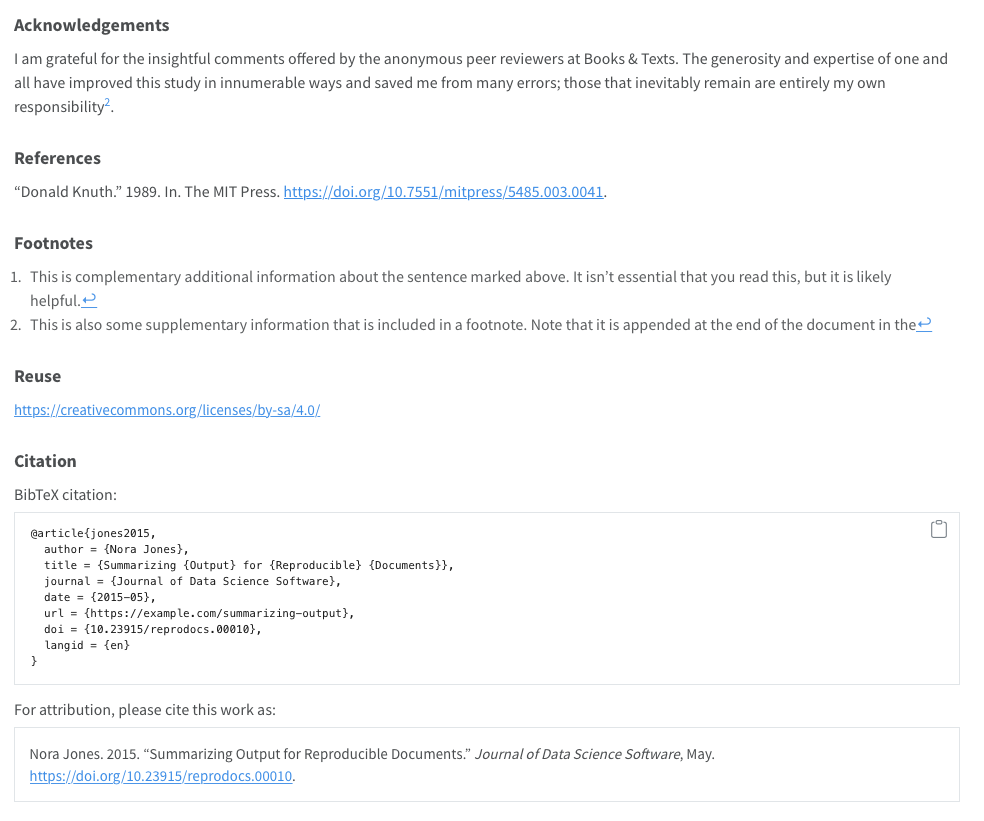The image features a clean, white background with distinct sections of text displayed in black print. At the top of the image, a header reads "Acknowledgments," followed by a statement of gratitude: "I am grateful for the insightful comments offered by the anonymous peer reviewers at Book and Text. The generosity and expertise of one and all have improved this study in innumerable ways and saved me from many errors. Those that inevitably remain are entirely my own responsibility."

Below the acknowledgments, the text transitions into the "References" section. Further down, a footnote area is indicated, followed by a "Reuse" section that includes a clickable website link. Next, the "Citation" section is presented, containing a detailed paragraph labeled "BibTeX Citation." This paragraph includes specific information about the author, title, journal, date, URL, and DOI.

At the bottom of the image, there is a "Language" section, and near the very lower part, a statement for attribution reads: "For attribution, please cite this work as:" which is contained within a rectangle. The citation inside the rectangle references Nora Jones, 2015, and her work titled "Summarizing Output for Reproducible Documents." At the bottom, there is another clickable link displayed in blue.